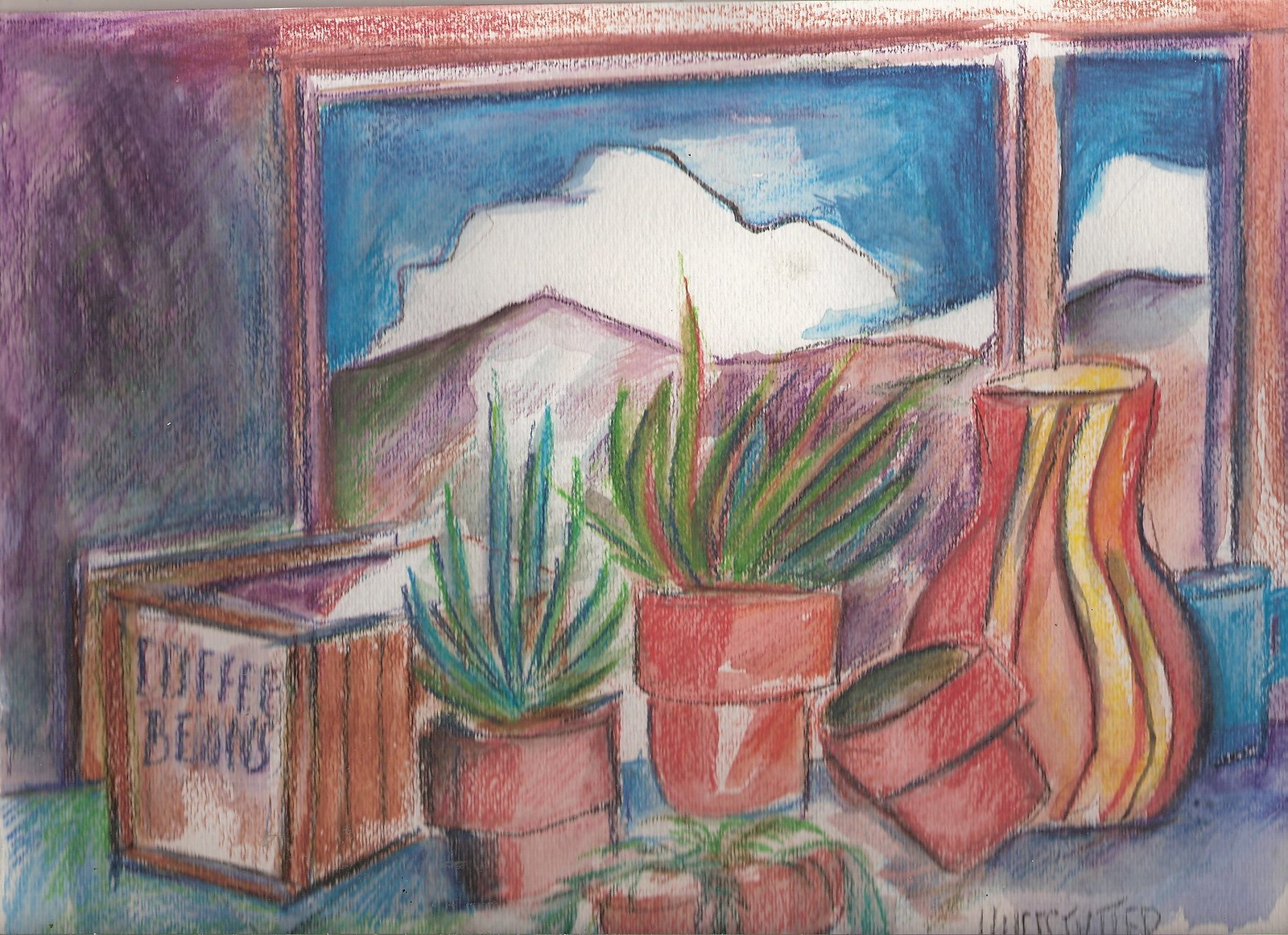This detailed artist's rendering, possibly created using chalk or pastel mediums, presents a serene view through a segmented window. The window features a wide left pane and a narrower right pane, both framed in a rich brown wood. Outside the window, a picturesque scene unfolds with a gently sloping hill beneath a sky adorned with fluffy white clouds on a clear, blue day. The interior wall, bathed in a soft purplish hue, adds a warm backdrop to the scene.

At the bottom of the painting, a countertop or shelf, laden with diverse pottery items, commands attention. Various plant holders and vases, filled with greenery, bring life and color to the composition. A wooden box labeled "truffle beans" sits prominently on the left, accompanied by three or four other potted plants, contributing to the cozy, rustic charm of the setting.